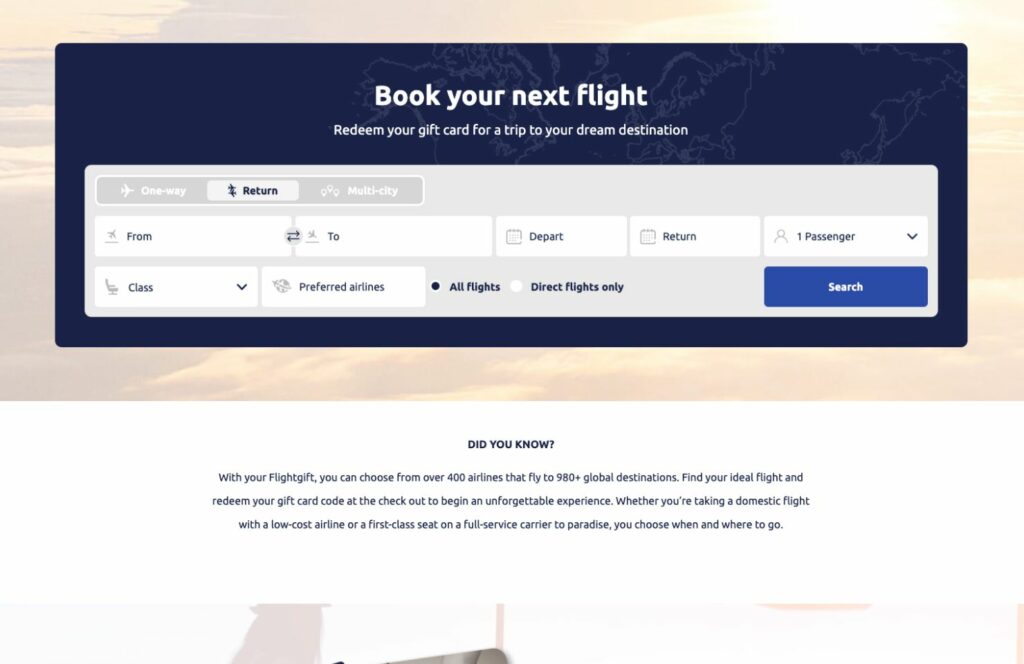Centered on a blue background, the website boldly displays "Book Your Next Flight" in white text. The background subtly features faint squiggly lines that resemble a map, adding a sense of adventure. Below the main message, the text "Redeem Your Gift Card for a Trip to Your Dream Destination" is also centered, written in a smaller font.

Nestled within the blue background is a grayish-white rectangular section. At the top of this section, there are options for "One Way," which includes an image of a plane, "Return," and "Multi-City." The next line displays input fields labeled "From," "To," "Depart," "Return," and "One Passenger." The following line prompts selections for "Class," "Preferred Airlines," "All Flights," and "Direct Flights Only." To the far right of this section, there is a prominent "Search" button in white text on a blue rectangle.